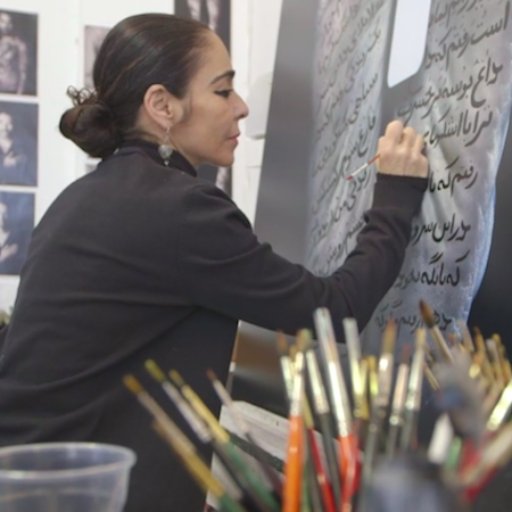This square color photograph captures a meticulous scene of a female artist engaged in calligraphy. She is positioned in front of a large easel, attentively working on a sizeable canvas adorned with delicate letters that appear to be Hebrew. The artist's hair is neatly tied back in a bun, allowing her to focus intently on her artwork. She is dressed in a dark hoodie or sweatshirt, contrasting with the silver or grayish background, which may be a piece of fabric draped over the canvas. The lower right corner of the image contains a slightly blurred group of paintbrushes of varying sizes and shapes, suggesting a dynamic workspace. Additionally, a clear plastic bowl or cup is positioned at the bottom of the image, possibly holding water or other supplies. The overall ambiance of the photograph is characterized by a dark, unobtrusive background that emphasizes the artist and her intricate work.